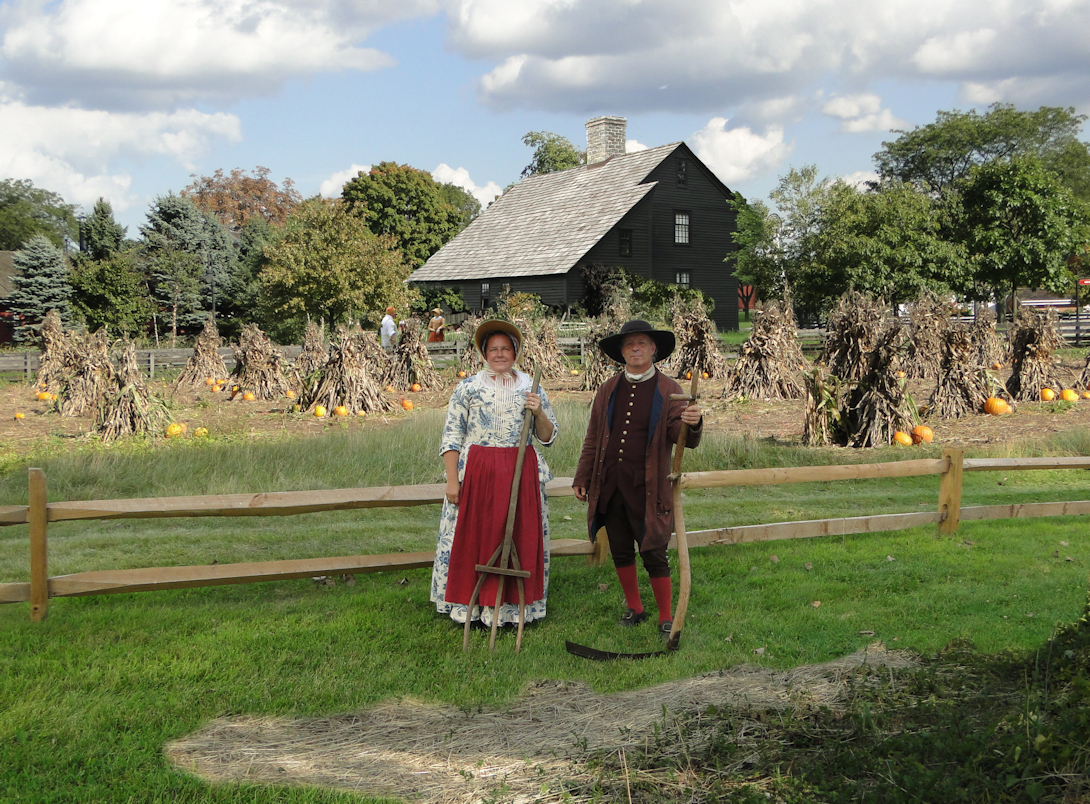In this photograph, a middle-aged couple stands in a pumpkin farm, dressed in pilgrim-like, centuries-old attire, possibly for a reenactment. The woman, positioned on the left, is adorned in a long, white floral dress with a red apron and bonnet, and she clutches a large wooden pitchfork. The man, on the right, dons a dark brown, long coat with gold buttons, brown knicker-style pants, red socks, and black shoes. He wears a wide-brimmed black hat and holds a full-length scythe. Behind them, a wooden fence encloses a field scattered with pumpkins and piles of dried hay or leaves. Further back, a dark gray house with a single top window stands against a backdrop of numerous trees and a cloudy sky.